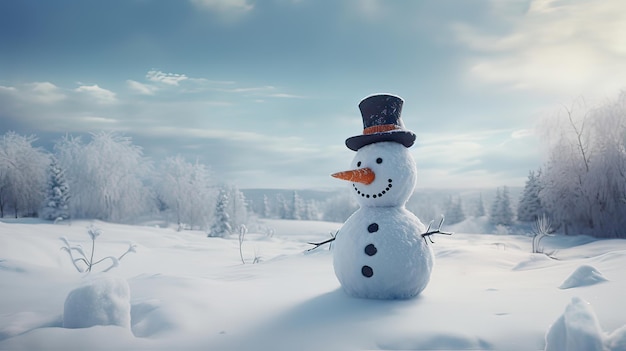This photo captures a serene outdoor winter scene during the daytime, with the ground blanketed in a thick layer of snow. At the center stands a cheerful snowman, composed of a large snowball for its body and a slightly smaller one for its head. It is adorned with a classic black top hat featuring a wide brim and a red ribbon. The snowman's face has two black rocks for eyes, a broad smile made of small black stones, and a prominent pointed carrot for a nose. Its arms are made of thin branches extending outwards. Three large black rocks are placed vertically on its belly, mimicking buttons.

In the foreground, the bottom right and left corners of the image show vast expanses of sparkling snow. To the left side, a small, Y-shaped tree or plant peeks out from the snow. The mid-ground is dotted with a mix of evergreen trees and possibly deciduous trees, all coated in snow, creating a picturesque winter landscape. The background features a row of snow-covered evergreen trees, adding depth to the scene. The sky above is a crisp blue, interspersed with fluffy white clouds, ranging from heavy to light and wispy, giving the entire setting a magical, frosty feel. No text is present in the image, emphasizing the tranquil beauty of the winter day.